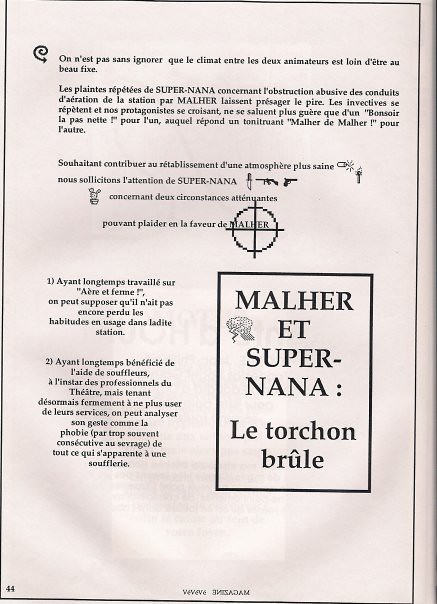The image depicts page 44 from a French book or possibly a journal, containing extensive text and symbols. At the top, an arrow symbol is present beside the line, "ONN'EST PAS SAN IGNORER QUE LE CLAMAT ENTRE LES DEUX ANIMATEURS EST LOI D'TRE AU," followed by the next line reading "BEAU FIXE." The page continues with several paragraphs of dense French writing. Throughout the text, there are various small icons including knives and guns pointing in different directions. In the lower section, the content is organized into two columns, with lists marked by numbers 1 and 2, possibly indicating poetic or journalistic entries. At the bottom of the page, a bold box contains large black text stating "M-A-L-H-E-R," followed by "E-T" and "S-U-P-E-R DASH N-A-N-A;" then another line reading "T-O-R-C-H-O-N BRULE." The page appears to have been scanned, with remnants of another page visible on the right edge.